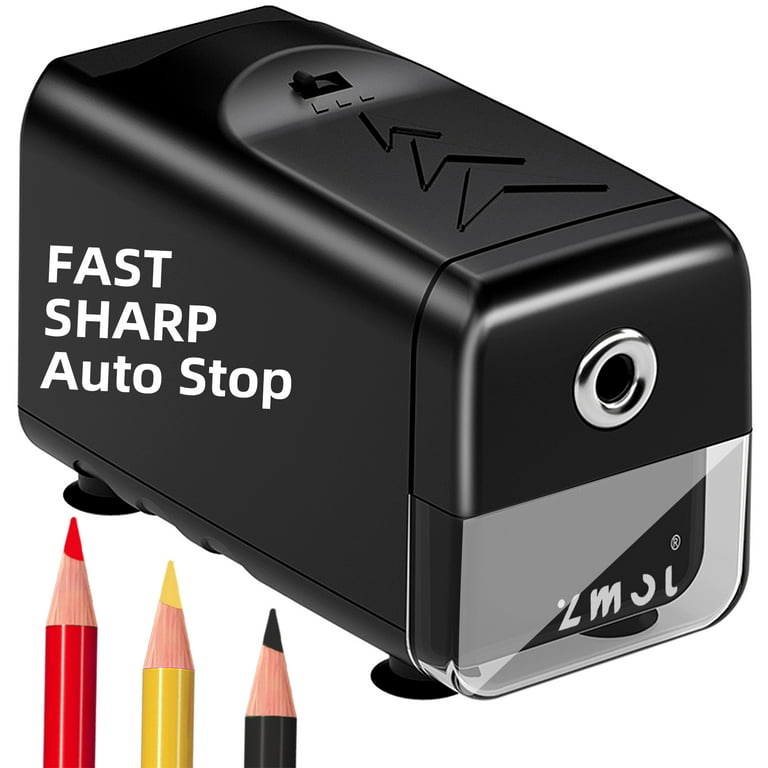This image showcases a black, plastic encased, electric pencil sharpener positioned at an angle towards the bottom right corner. The pencil sharpener is rectangular in shape and prominently features a silver metal opening where pencils are inserted. Below this opening is a transparent compartment that allows visibility of the pencil shavings and has the brand name "ZMOL" printed on it in white text. Additionally, the left side of the sharpener displays the text "Fast Sharp Auto Stop."

On the top of the sharpener, there are three arrows arranged in an oval pointing towards a protruding switch that controls the sharpening settings. At the bottom, the sharpener is supported by legs equipped with suction cups or grippers to keep it stable on a surface. In the bottom left of the image, three colored pencils—red, yellow, and black—are shown at varying levels of sharpening, providing a reference for the sharpener's functionality.